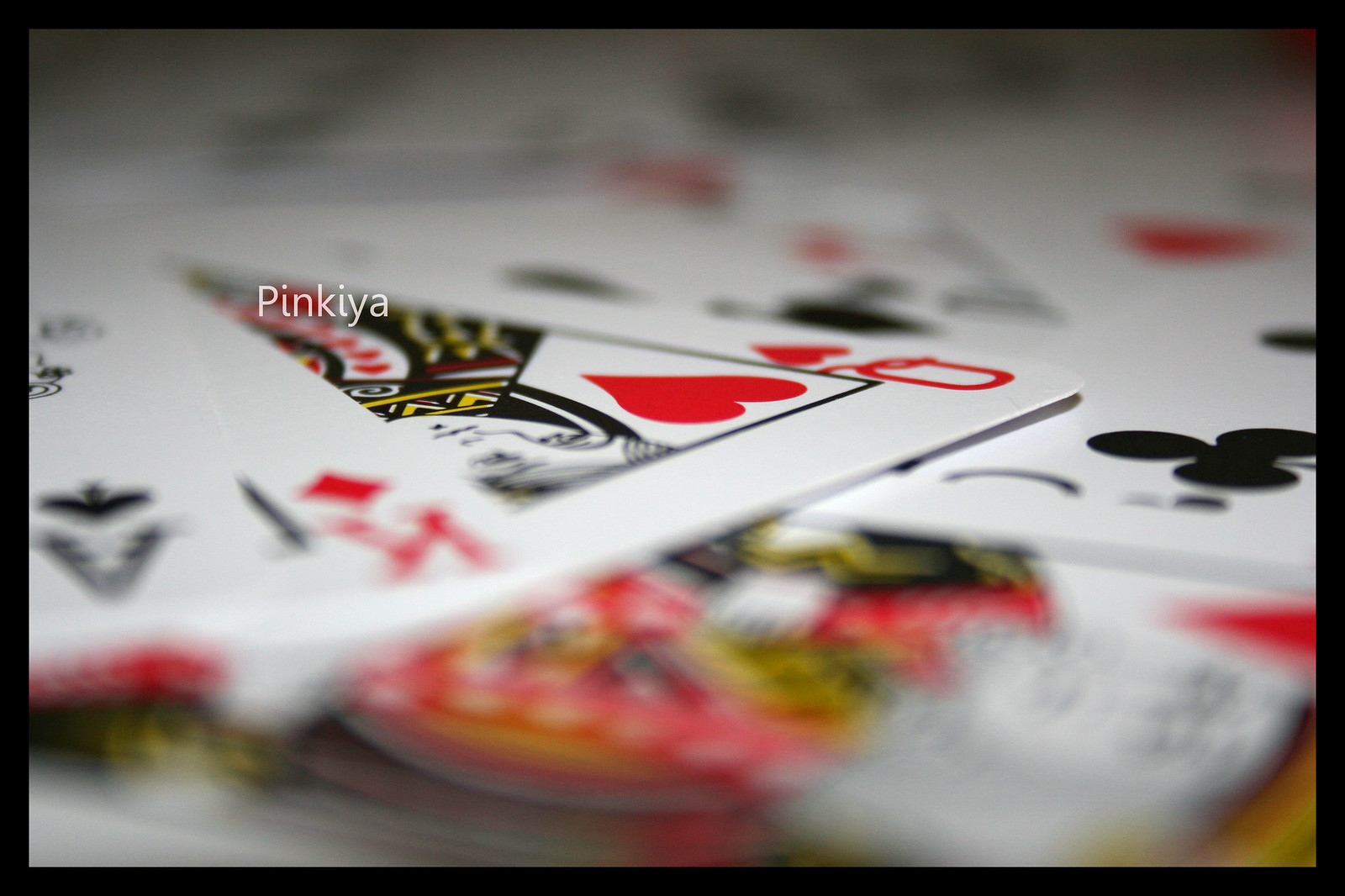The image portrays a dynamic arrangement of playing cards, shuffled into various positions, with a notable display of reds, blacks, and a touch of yellow. At the top of the image, a prominently featured Queen of Hearts card stands out. This card is predominantly white, showcasing a queen dressed in a striking yellow and black outfit. A large red heart adorns the side of her face, outlined in black, which is placed within a red-bordered square. Below this square is another red heart symbol. In the background, partially visible and slightly blurred, is a King of Diamonds card indicated by a "K" and its corresponding red diamond symbol. Additionally, an Ace of Spades card is discernible with an "A" and a spade symbol. Just beneath the Queen of Hearts, a black club symbol is also visible. Although the image is blurry towards the bottom, the overall composition is vibrant with the interplay of red, black, and yellow hues, creating a visually engaging ensemble of shuffled playing cards.